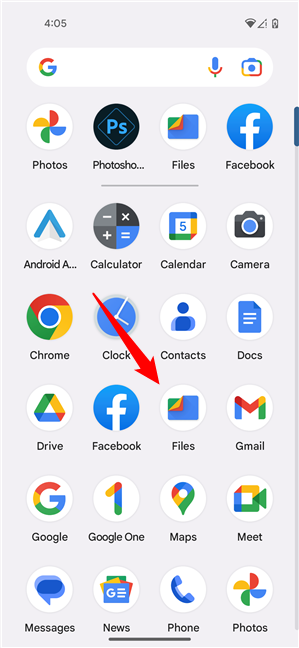This image showcases the Android app drawer, a centralized hub displaying all installed applications. The app icons, predominantly circular, include Photos, Photoshop, Files, Facebook, Android Auto, Calculator, Calendar, Camera, Chrome, Clock, Contacts, Docs, Drive, Gmail, and Google. Notably, some applications appear twice, such as Files, Facebook, and Photos. An arrow has been added to highlight the duplicated Files app, prompting curiosity about the redundancy. The light grey background contrasts with the app icons, many of which feature shades of blue. The orderly arrangement and color scheme exemplify the typical Android interface, but the presence of duplicate apps adds an unusual and intriguing element.